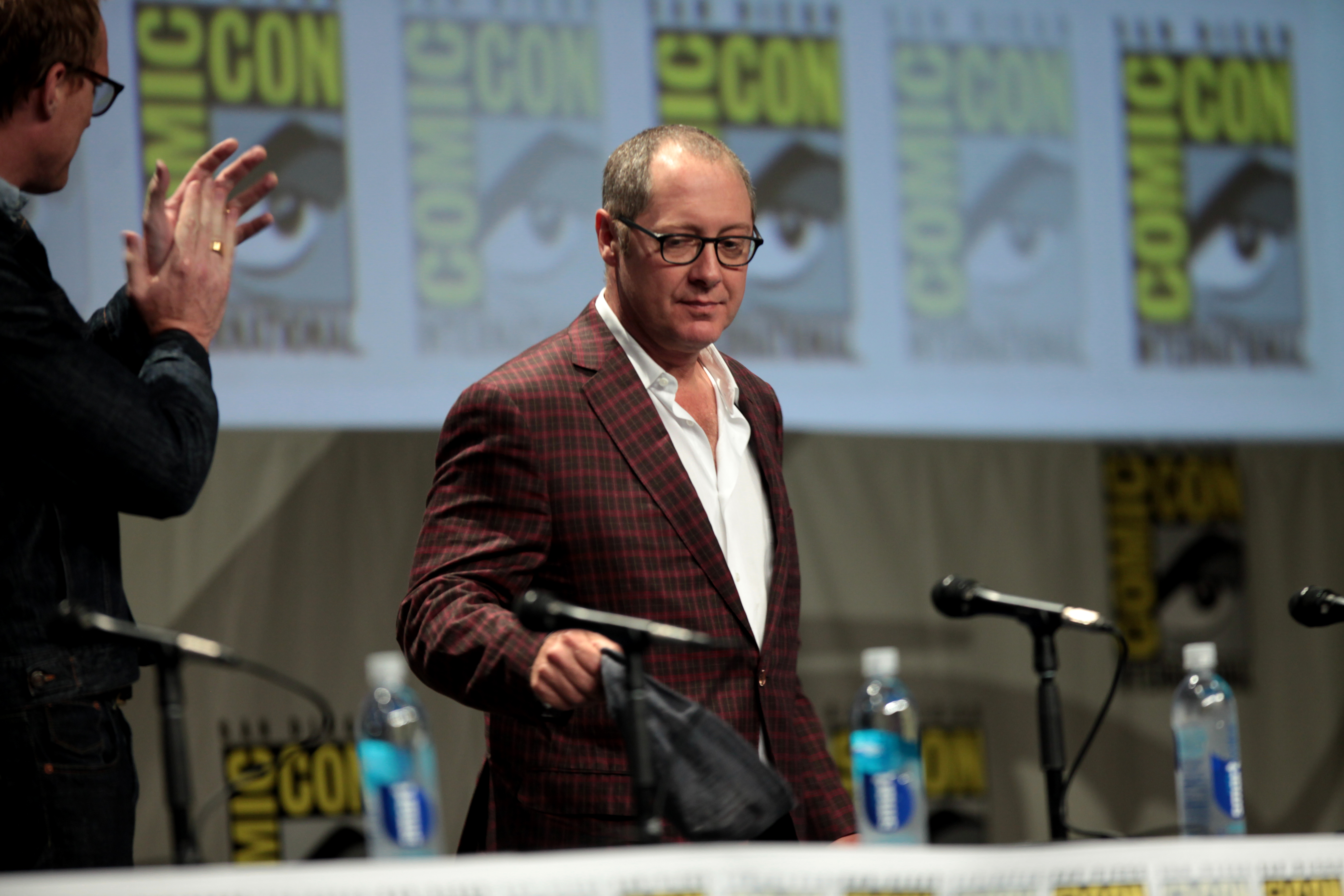The image captures a Comic-Con panel set against a backdrop of pale blue and gray, adorned with vertically aligned Comic-Con posters, each featuring the words "COMIC CON" in bold yellow letters and a serious-looking eye illustration. The main focus is on a long rectangular table in the foreground, draped with a white tablecloth, hosting four black microphone stands with corresponding microphones, three of which are attended by flexible black wires. Alongside the microphones sit three clear plastic water bottles with white caps.

At the table, two men are present. The man in the center, visible from the waist up, sports a sharp black and green plaid jacket over a white button-up shirt with the top three buttons undone. He wears black-framed glasses and appears to be slightly stout, looking downward with his right arm bent at the elbow. The man to the left, partially cut off by the image's edge, is captured in a side profile. Dressed entirely in black with a long-sleeve shirt, black pants, and black-rimmed glasses, he seems to be clapping, revealing a gold ring on his right ring finger.

The background showcases a repetitive series of Comic-Con posters, adding a unified yet vibrant touch to the scene. The setting and visual cues suggest a formal yet engaging atmosphere, typical of a Comic-Con panel presentation.